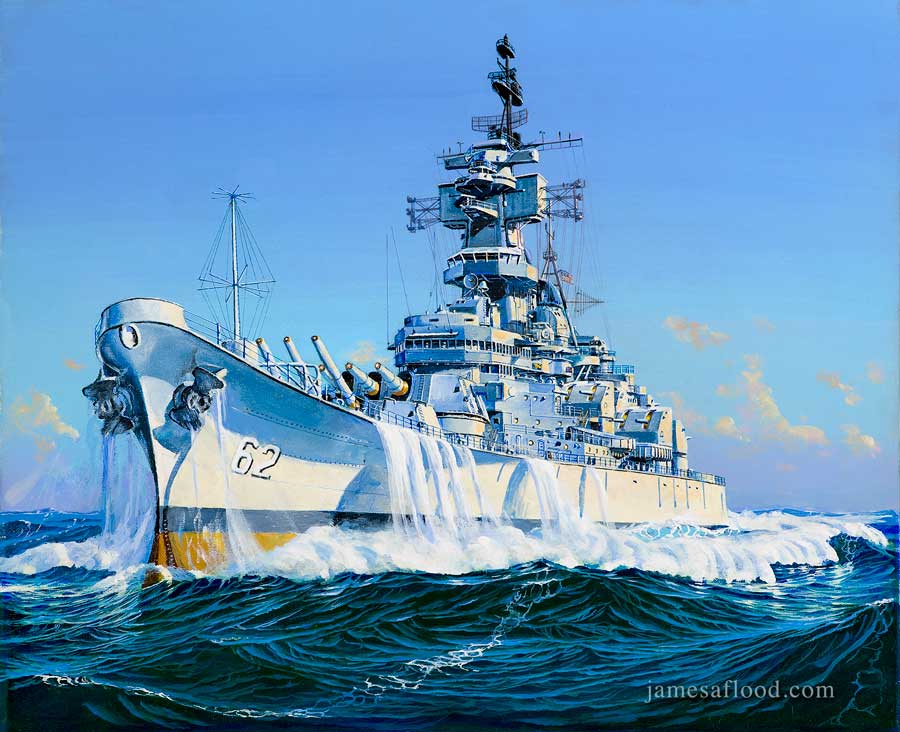This image depicts a digitally rendered painting of a large warship navigating a calm ocean under a clear, sunny blue sky that occupies two-thirds of the scene. The ocean at the bottom third is a deep blue, with visible waves gently lapping against the ship. The warship, marked with the number 62, features multiple decks and levels adorned with numerous radars, antennas, and missile guns pointing forward. The ship, angled at a 45-degree orientation from the viewer's perspective, exhibits a prominent white upper deck with horizontal stripes of blue and yellow below. Cascading waterfalls of seawater can be seen flowing off the sides of the ship. The image bears the watermark "jamesaflood.com" in the bottom right corner, suggesting the artist behind this intricate and vibrant depiction.